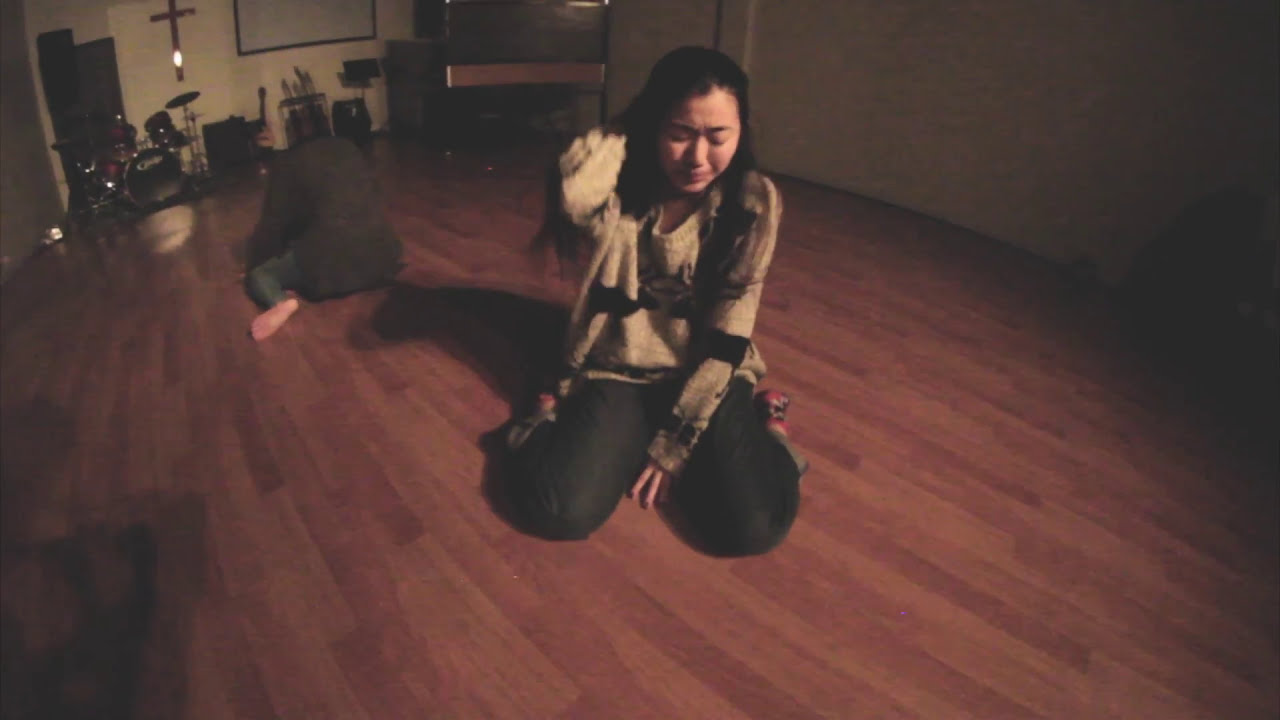In the center of a small, shadowy room with beige walls and a brown wooden floor, a Chinese woman with black hair is sitting on her knees, looking distressed and likely crying. She is wearing dark pants and a beige sweater with a black strap across it. Her eyes are closed, and one arm is behind her head. In the background of the room, there is a cross on the wall, a drum set below it, and a guitar with some amps to the right. Another person, also barefoot and with their head down, sits in a similar position behind her. The overall scene suggests a moment of emotional intensity, perhaps during a private or religious gathering.